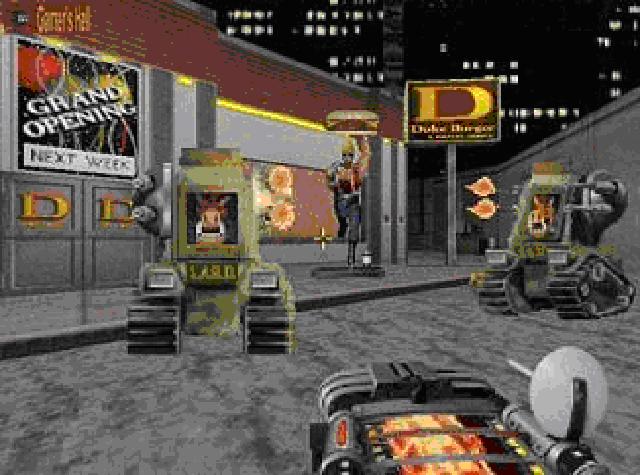This detailed screenshot from a video game presents a lively, animated city street scene, depicting two green, military-styled vehicles with large wheels, seemingly driven by whimsical characters resembling a rabbit or donkey. The game adopts a first-person shooter perspective, as indicated by a small gun-like object protruding at the bottom front of the screen. Centered in the background, there's a statue of a character triumphantly holding a hamburger above its head, adding a humorous touch. Nearby stands a prominent sign with a big yellow "D," believed to be advertising "Duke's Burger," even though the text underneath is partially illegible. Additionally, a large "Grand Opening Next Week" banner is displayed, suggesting a new store about to launch. The backdrop includes buildings with illuminated windows, contributing to the vibrant city atmosphere. Another smaller figure, resembling a soldier in a gray uniform with orange and red accents, appears near the vehicles, poised with an arm extended. This chaotic yet colorful scene contrasts the detailed military vehicles with the playful, cartoonish elements and bright city street setting.